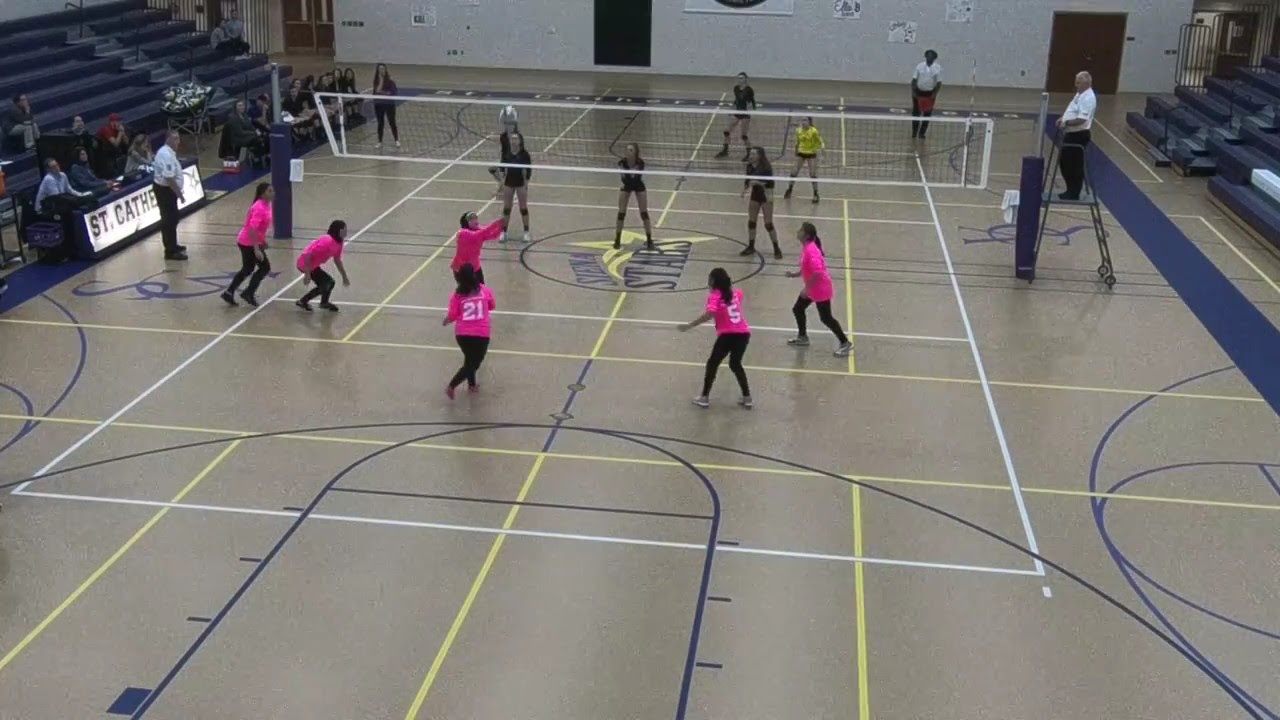The image captures an intense middle school girls' volleyball match inside a gymnasium. On one side, the team is outfitted in black pants and bright pink jerseys with white numbers, including a player wearing jersey number 2 and another in jersey number 5. Opposing them, the second team sports black shorts and black jerseys, with one standout player in a yellow shirt. This action shot features the volleyball in mid-air, headed toward the pink team, where a player appears poised to set it up for a spike. The gym's tan flooring is marked with blue, yellow, and white boundary lines, indicative of various play areas. Visible in the background is a white wall adorned with several sets of brown doors fitted with silver push bars. Scattered spectators occupy the stands, along with referees and coaches positioned along the sidelines. A scorekeeper can also be seen tracking the game, along with a lighted sign that reads "St. Catherine's."